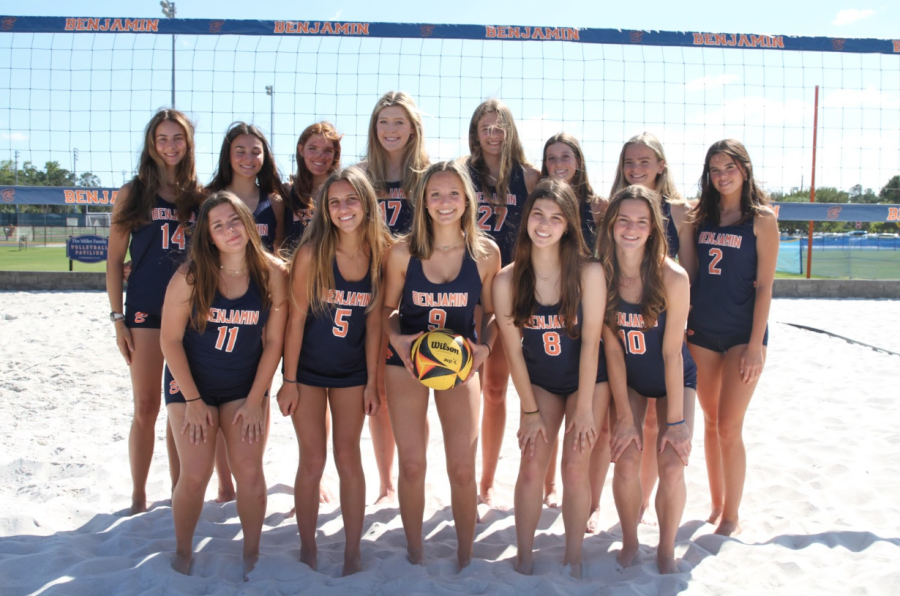This photo captures a high school girls' beach volleyball team posed cheerfully in the sandy playing area of a volleyball court on a sunny day with clear skies. The team, consisting of 15 girls, is grouped in two rows—eight in the back standing and seven in the front kneeling. Each girl wears a navy or black volleyball uniform adorned with "Benjamin" and their individual numbers in orange outlined with white. They stand in front of a volleyball net with blue outlines and "Benjamin" repeated in orange across it. The girl at the center prominently holds a yellow and black Wilson volleyball, its brand logo clearly visible. In the background, the scenery hints at possible school fields or a park, adding to the open and vibrant atmosphere of the photograph.